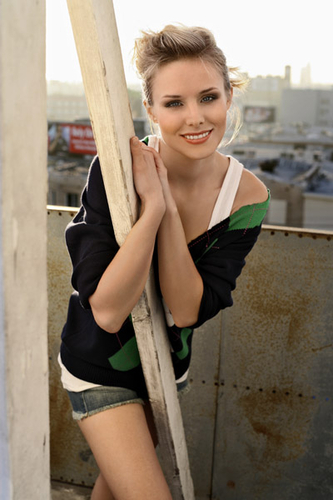The photograph features a young Caucasian woman, who appears to be actress Kristen Bell, posing with a smile. She has blonde hair styled in a high, poofy bun and wears a notable amount of eyeshadow and mascara. Her attire includes a white tank top beneath an off-the-shoulder black hoodie with green accents, and she pairs this with denim short shorts. The woman, who has light skin and red lipstick, stands with her arms wrapped around a green-colored, triangular steel beam, giving a slight leftward lean while tilting her head slightly to the right. The setting includes a rusted metal wall adorned with visible rivets that reaches up to her mid-back, and a cityscape in the background, indicating she’s at an elevated position. Bright light illuminates her, drawing attention to her cheerful demeanor and detailed features.